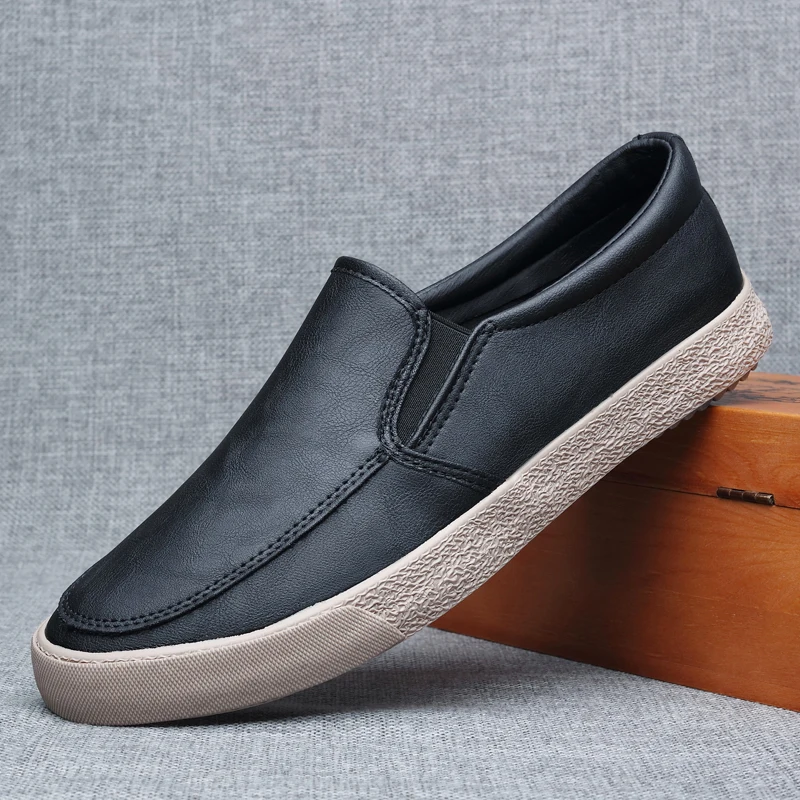The photograph showcases a comfortable black slip-on tennis shoe, perfect for both casual and office wear. The shoe features a stretchy tongue for easy slip-on, complemented by black topstitching and a textured, padded foam ring around the ankle for added comfort. The upper part, made of what appears to be black leather, includes an elastic insert to ensure a snug fit. The shoe's bottom is crafted from tan-colored rubber with visible nubs of tread on the heel, enhancing its safety and traction. Its front toe is protected by stippled rubber, while the back has a grainy texture for durability. The shoe is propped up on a dark brown wooden box with gold hinges, which lies atop a gray fabric background. The box provides an angled support, elevating the heel while the toe rests on the ground, creating an appealing display likely intended for an advertisement.